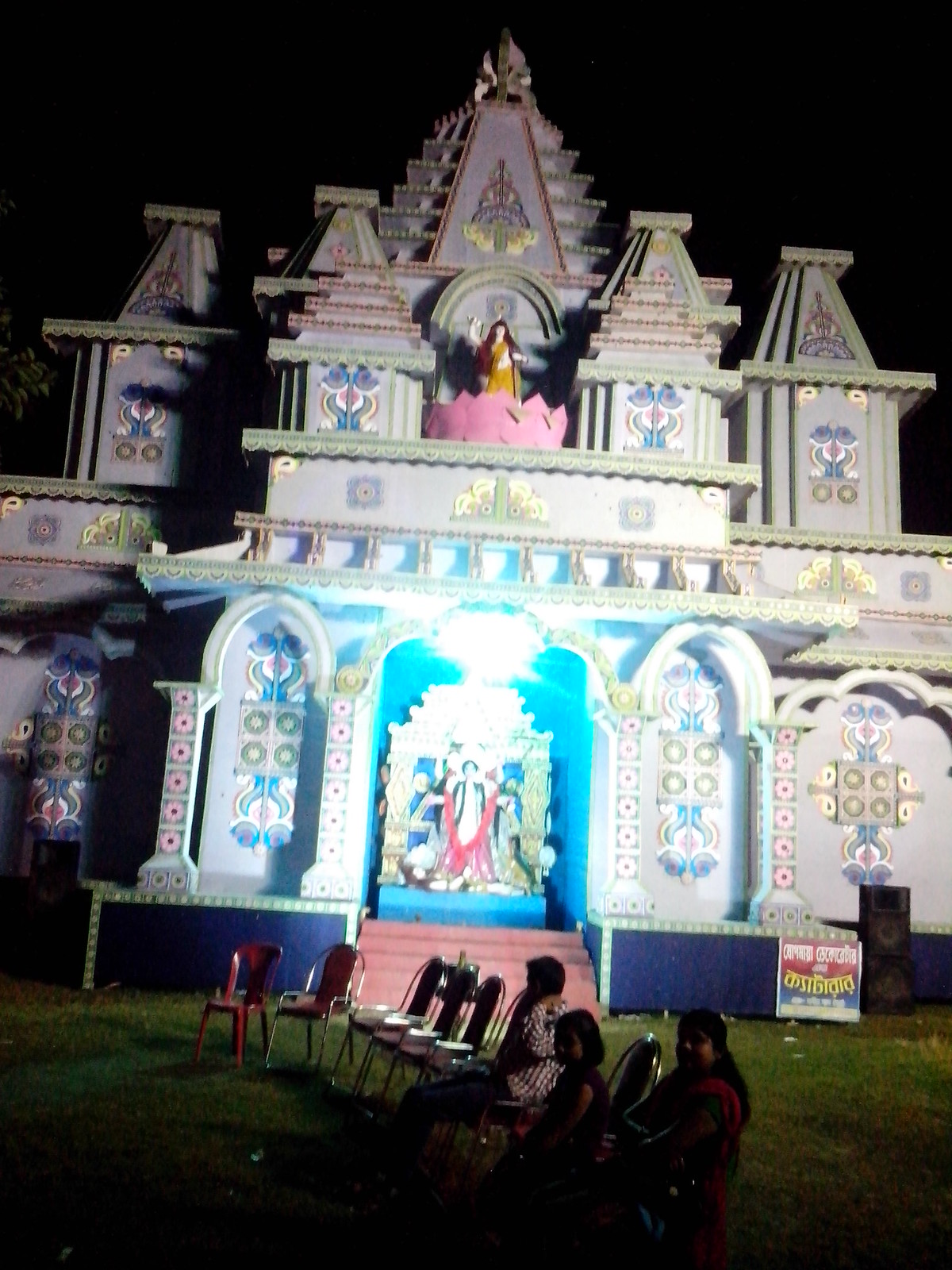The photograph is a vertical, rectangular color image taken at night, featuring an ornate building that resembles a Hindu temple or an elaborately decorated castle. The sky is pitch black, accentuating the artificial lights illuminating the scene. In the foreground, three individuals are seated on chairs placed on dark green grass. The building, painted in white with blue trim and featuring multicolored, finely decorated pillars, is approximately two stories tall. 

At the base, there are several archways with an ornate wall underneath. A staircase leads up to the entrance, where a painting of a person stands, bathed in light. Above, the structure is crowned with several pointed triangles or spires, decorated in gold. In the center, a statue of a girl wearing a yellow sari stands within a pink flower, placed prominently for all to see. The foreground features a sign on the grass, though the text is unreadable. The scene is meticulously illuminated, highlighting the details of this captivating nighttime outdoor setting.